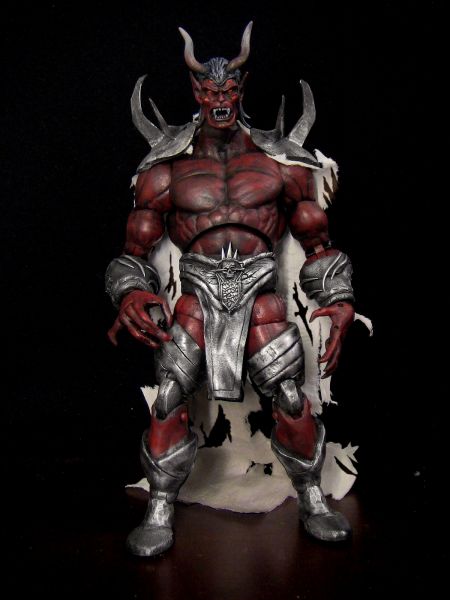The image depicts a highly detailed fantasy action figure standing on a wooden table with a black background. This devilish warrior character is strikingly muscular with a vividly dark red body, a defined chest, and a chiseled stomach. He exudes a menacing presence with his sharp, large fangs and fierce red eyes, his mouth agape in a vicious snarl. His head is adorned with a metal helmet featuring imposing horns, crafted from a pewter-like material rather than shiny silver.

The figure is clad in comprehensive silver metallic armor: boots, underwear, rings around his upper legs and lower arms, and shoulder guards that boast several sharp spikes. His wrists are also encircled with metallic armor, and his hands are exaggeratedly large with elongated, claw-like fingers. Around his waist, there is a skull and a piece of cloth, contributing to his fearsome appearance. Adding to his formidable look is a tattered white cape or cloth draped behind him, further enhancing the fantasy aspect of this intricate figure.